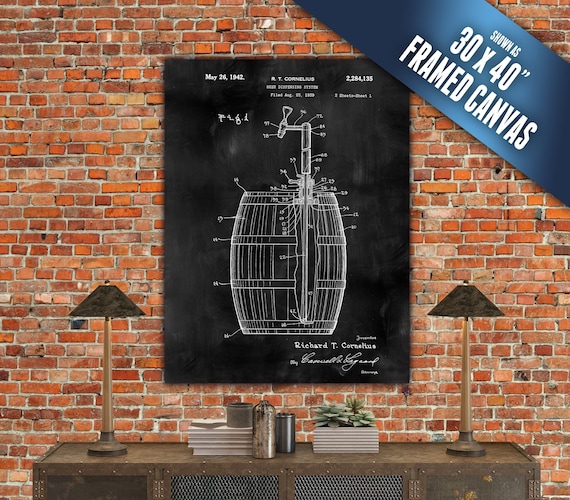The image depicts a detailed scene featuring a red brick wall with a blackboard mounted on it, creating a striking contrast. The blackboard, which has a chalkboard effect, showcases a white diagram resembling a blueprint or patent drawing of a barrel with a spout, possibly used for alcohol. The diagram includes several numbers and the text "May 26, 1942," along with the name "Richard T. Cornelius" at the bottom, suggesting it might be a historical patent. In front of the brick wall, there is a wooden table adorned with various items including lamps on either side, books, vases, and succulent plants. Above the scene, in the top right corner, there is diagonal text that reads "shown as 30 by 40 framed canvas," indicating the dimensions of the artwork. The rich details and vintage elements combine to create an evocative and historic atmosphere.